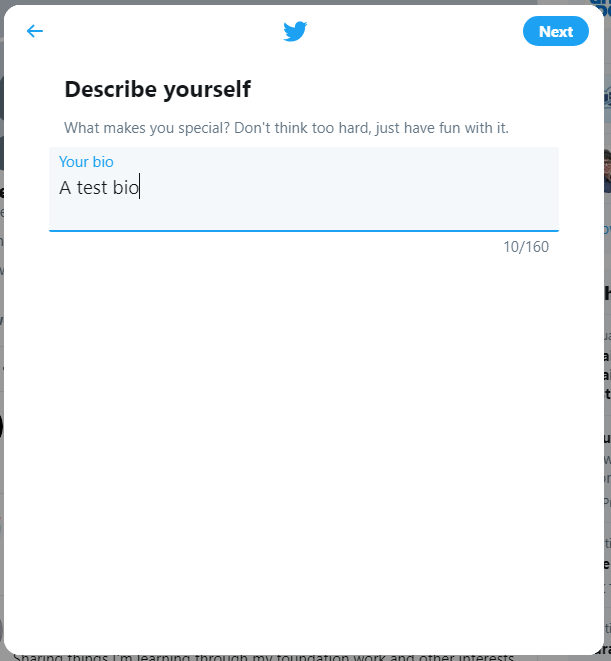The image shows a white rectangular overlay partially obscuring another image, with fragmented text visible on both the left and right edges of the underlying image. In the top-left corner of the overlay, a blue arrow points to the left. Centered below the arrow is the Twitter icon featuring the signature bird. To the far right, there's a blue button labeled "Next."

Beneath this navigation area, the instruction "Describe yourself" appears in bold black text, followed by a smaller gray prompt that reads, "What makes you special? Don't think too hard; just have fun with it." Below this, a light blue box is labeled "Your bio" in blue at the top. Inside this box, gray text reads "A test bio." A dark blue line runs along the bottom of this area, marking the end of the text field.

In the bottom right corner, it says "10/160," indicating the character count of the bio. The rest of the image is filled with blank white space.